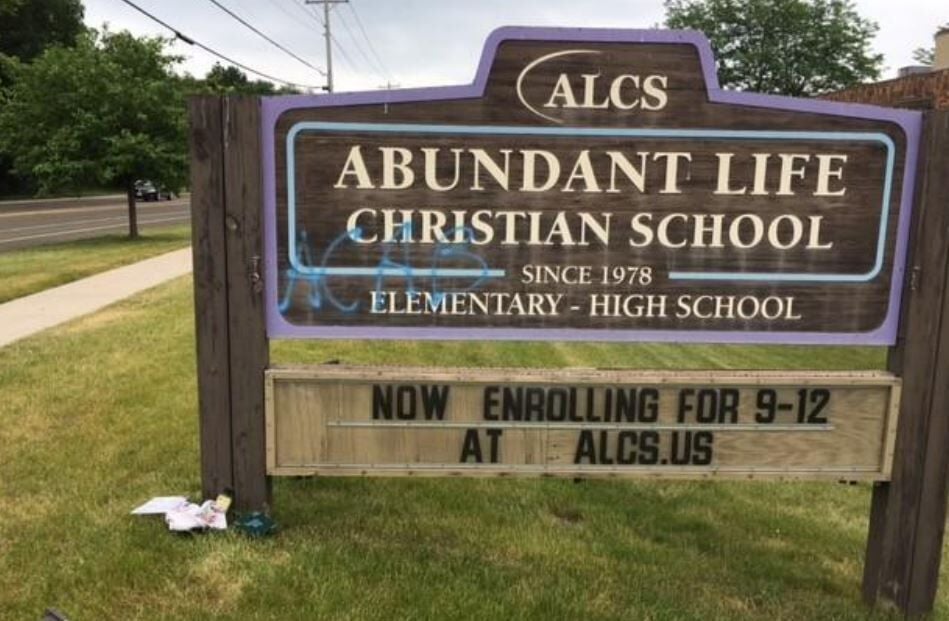This is an image of a weathered wooden sign standing prominently in front of Abundant Life Christian School (ALCS), established in 1978. The sign, trimmed in purple and bearing white letters, is positioned atop fresh mulch and surrounded by green grass. It prominently displays the school's name and the message: "Now enrolling for 9-12 at ALCS.us." There is notable blue graffiti on the sign, with the letters ACAB, hinting at possible local tensions. Scattered litter lies near the sign, and a sidewalk and a passing car can be seen in the background, accentuating the sign's roadside placement.